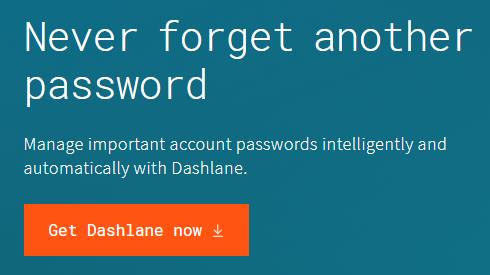The screenshot depicts a promotional banner from a website. The rectangular banner, which is slightly wider than it is tall, features a deep blue or bluish-gray background. 

In the upper portion of the banner, large white text spans across the width, stating "Never forget another password." Below this, an indented line reads "Password," also in large white letters. 

Further down, smaller white text offers additional details: "Manage important account passwords intelligently and automatically with Dashlane," with the last part also indented to the left.

At the bottom left of the banner, an orange rectangular button stands out, containing the call-to-action "Get Dashlane now" in white text. Just to the right of this button, there is a download icon—a downward arrow with a horizontal line at the bottom—likely serving as a quick link to download the application.